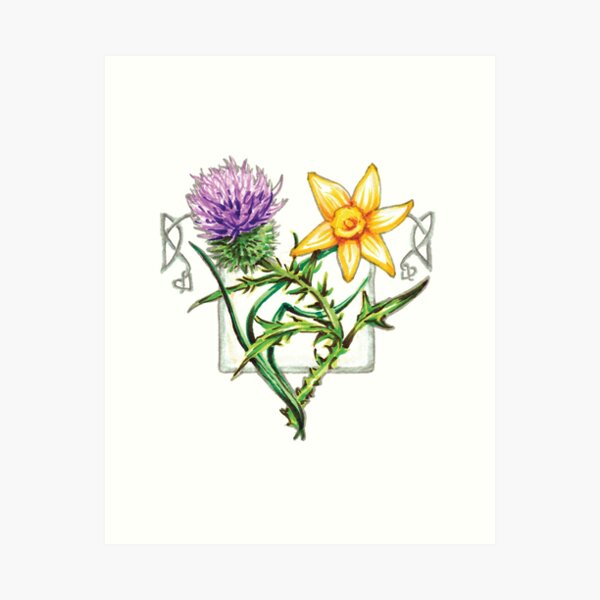This is a detailed drawing, reminiscent of an old-fashioned seed packet or farmhouse style illustration, featuring two intertwined flowers on a white background. The flowers are framed by a light blue border forming three sides of a square. To the left and right of the flowers, there is a scrolling design, somewhat heart-shaped, done in a silvery-blue color, giving the impression of delicate, looping wire.

The flower on the left is a thistle, characterized by a fluffy purple bloom and a spiky, light green stem. The flower on the right resembles a daisy with six yellow petals, attached to a smooth, darker green stem that winds toward the left and downwards. The overall artistry appears to be hand-drawn, possibly with colored pencils, giving it a cute and charming look despite its light detailing. The slight gray hue of the background contrasts subtly with the white, paper-like canvas, enhancing the floral imagery.